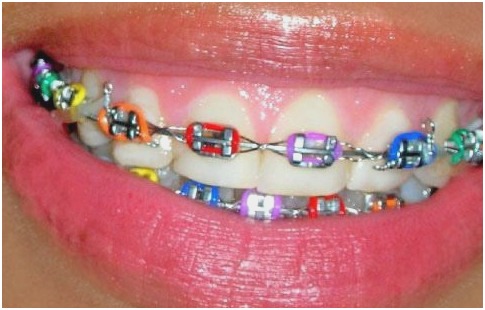This close-up photo captures a detailed look at a smiling mouth, showcasing both the teeth and lips. The lips, coated with pink lipstick, frame a set of braces-laden teeth. Each silver metallic brace is uniquely adorned with a colorful epoxy, arranged in a repeating pattern of green, yellow, orange, red, purple, and blue on both the top and bottom rows of teeth. The braces are characterized by H-shaped brackets. The off-white teeth suggest a natural, unbleached color beneath the vibrant, fun colors of the braces, which add an element of playfulness to this dental apparatus. The surrounding skin and gums share hues of pink, further enhancing the overall warm tint of the image. The person in the photo could be either a male or a female, but the details lean slightly towards a depiction of a female, given the pink lipstick.